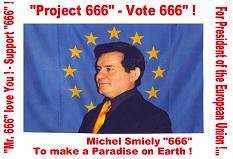The image is a horizontally aligned, rectangular screen grab of a campaign advertisement with a white background. At the center is a portrait of a man against a blue, banner-like backdrop adorned with yellow stars arranged in a circular pattern. The man, identified as Michael Smiley, is a white male with short, dark hair, wearing a dark suit jacket and a gold tie, and facing to his left with a closed-mouth smile. Above his image, in bold red letters, it reads, "Project 666 - Vote 666!" Vertically along the right side, also in red, it declares, "For President of the European Union!" On the left side of the advertisement, in red text, it states, "Mr. 666, love you! Support 666!" At the bottom, in red text, it says, "Michael Smiley '666' - To make a paradise on earth!" The text outlines the top, bottom, left, and right of the image, emphasizing the campaign’s central message and the candidate’s name.